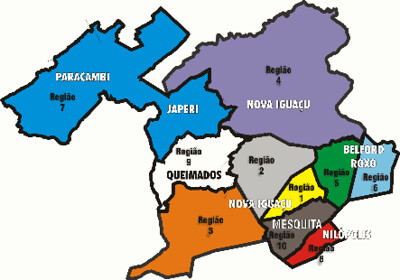This image is a detailed geography map depicting ten regional provinces, each distinguished by a unique color and numbered from 1 to 10. Starting with number 1 in yellow, number 2 in gray, number 3 in orange, number 4 in purple, number 5 in green, number 6 in light blue, number 7 in dark blue, number 8 in red, number 9 in white, and number 10 in brown, the map appears to represent sections of a specific country or region.

In the left section, labeled in blue, we see provinces named Jopiri and Parakamri, almost the largest areas. To the right, the purple-colored section is Nova Iguacu, notable for its expansive size by area. Below these, the white section is identified as Queimados. Adjacent to Queimados is a gray area, with a green section beside it, and a light blue section next to the green, labeled Belford Roxo.

The middle section features interconnected areas: the gray section has a yellow section beneath it, transitioning into a darker purple section, marked Mosquita, and then a red section labeled Nilopolis. Beside this region, there is a larger orange section lying to the left of the dark purple and beneath the white section, potentially part of Nova Iguacu based on color similarities.

Overall, this map, despite being in another language, effectively distinguishes these provinces through distinct color coding and labels, providing a visual separation of each regional area.